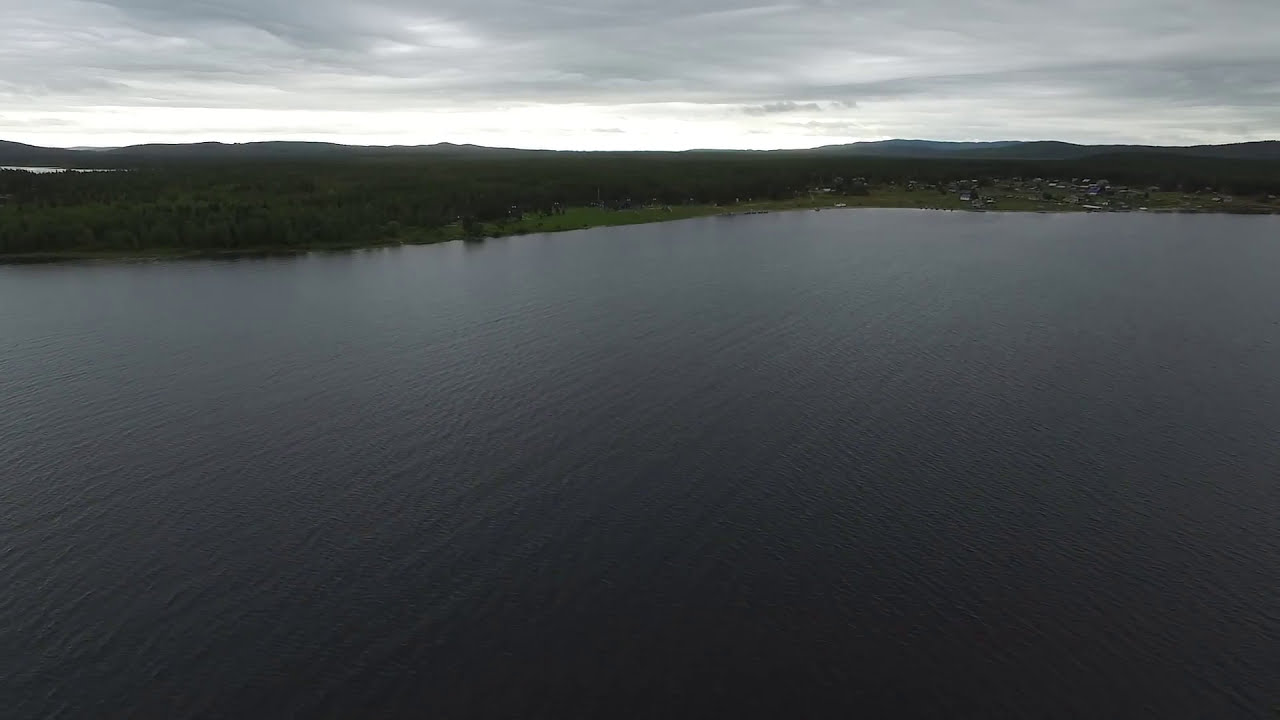The photograph captures a serene and expansive lake, occupying the lower two-thirds of the frame. The water's surface displays slight ripples, indicating a gentle breeze but no strong currents or disruptions from vehicles or people. In the upper third of the image, a dark silhouette of mountains or hills creates a striking contrast against the water, while an overcast sky with thick gray clouds looms overhead. The sun is hidden behind these clouds, casting a subtle glow on the horizon and enhancing the grayscale gradient of the scene. The entire image exudes a muted, underexposed atmosphere, with minimal color or detail visible due to the dense cloud cover. The landscape appears to be viewed from an elevated vantage point, looking towards a distant shoreline that is obscured and indistinct, suggesting the presence of greenery and possibly some housing developments, though specifics remain elusive in the dark, shadowy panorama.